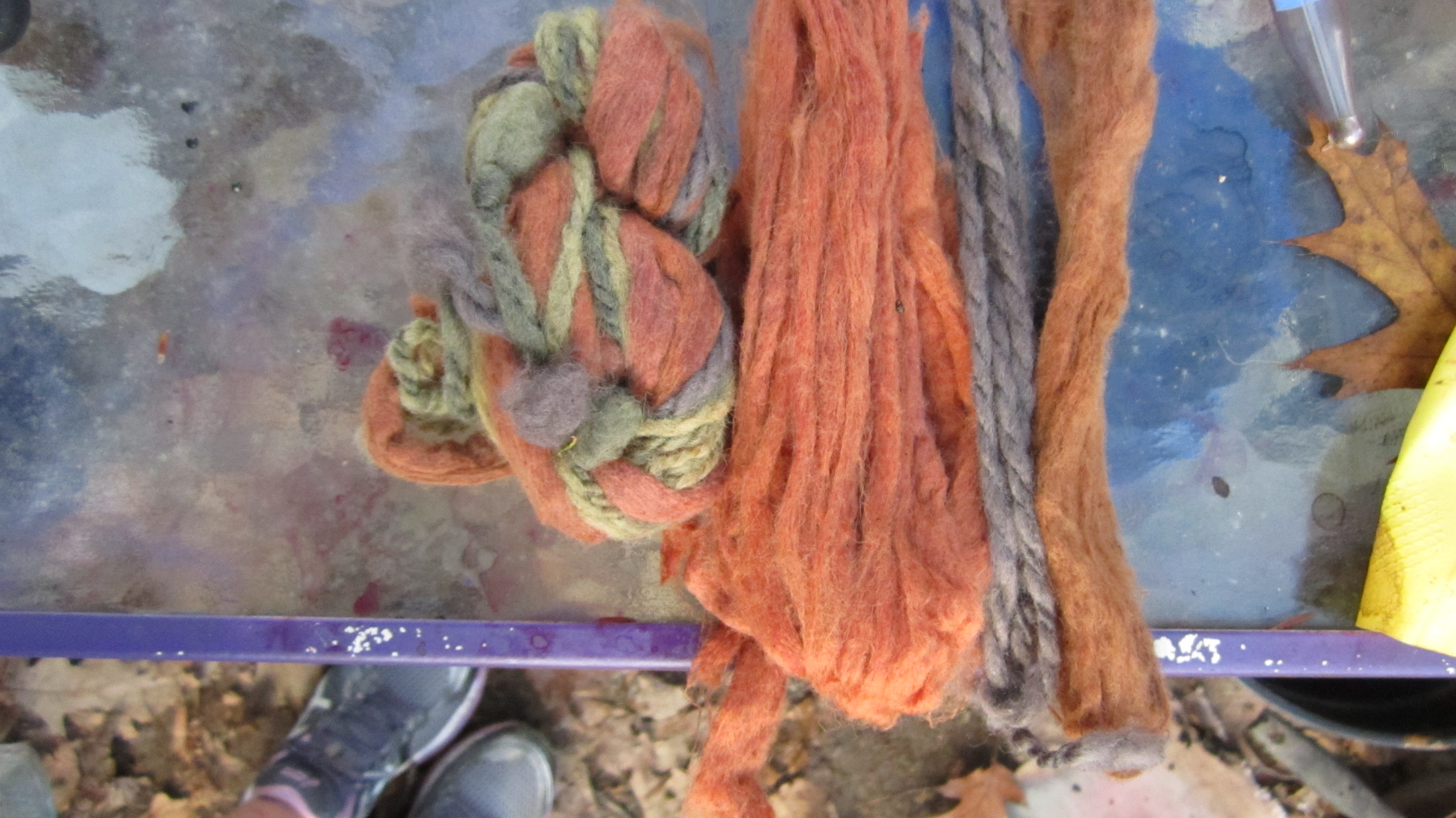In this close-up color photograph taken from above, a worn and tangled multi-colored ball of yarn—comprising red, gray, brown, orange, and gold strands—rests on a paint-splattered table with purple-painted trim. A large maple leaf sits prominently on the table's right side. The table appears to be a messy, possibly makeshift workstation, with scattered white specks adorning the purple edges. In the foreground, beyond the table edge, stands an individual on a dirty ground, their feet shod in black, pink-splattered tennis shoes. A large thermometer can be observed in the right corner. The scene, likely set in a construction site or an old decaying building, suggests an environment amidst cleaning or repair, featuring a mix of colors—gray, purple, and blue—beneath the tangled yarn.